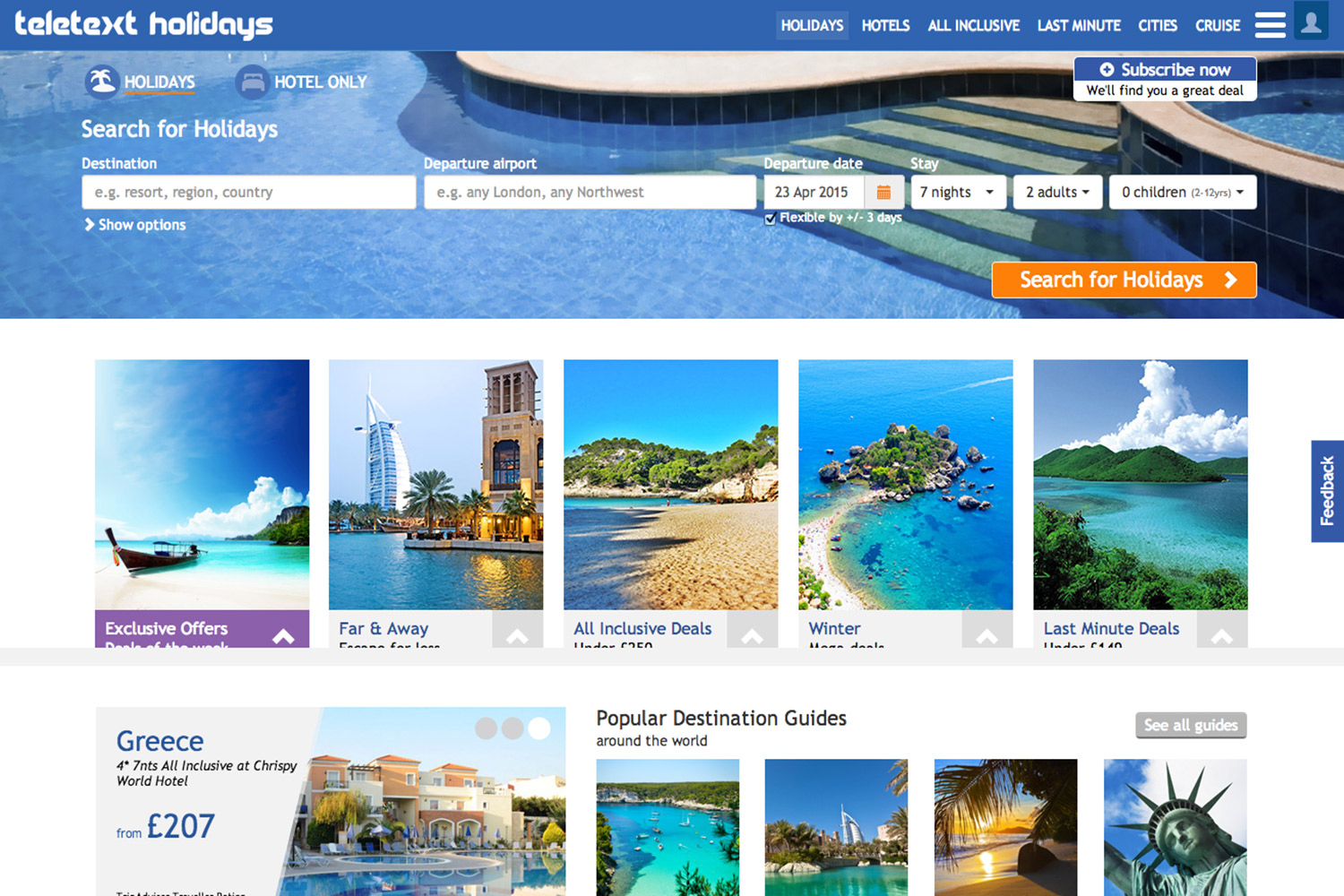The screenshot captures a web page layout for Teletext Holidays. At the top, a blue navigation bar spans the width of the page. In the top left corner, the Teletext Holidays logo is prominently displayed in white text. On the right side of this bar, several menu items are listed in white, including "Holidays," "Hotels," "All Inclusive," "Last Minute," "Cities," and "Cruises."

Directly below the navigation bar is a visually engaging section featuring a background image of a swimming pool. The pool's blue water is accentuated by steps that lead up to a curved walkway, contributing to a serene and inviting visual.

On the left side of this section, there are options to refine holiday searches: "Holidays," "Hotel Only," and "Search for Holidays." Beneath this are several input fields for customizing a search, including destination, departure airport, departure date, stay length, number of adults, and number of children. An orange button reading "Search for Holidays" stands out, inviting users to begin their holiday search.

Further down, the content area features a white background with a collection of destination images. The first image on the left showcases a picturesque beach scene with a boat anchored near the shore. Next to it, a waterfront scene includes a prominent white tower beside a brownish tower. To the immediate right is another scenic beach replete with golden sands and rolling hills adorned with green trees. The succeeding image depicts a clear blue sea, with a small island-like formation connected to a sandy shore. The final image presents lush, green rolling hills beside tranquil blue waters, capturing a sense of peaceful retreat.